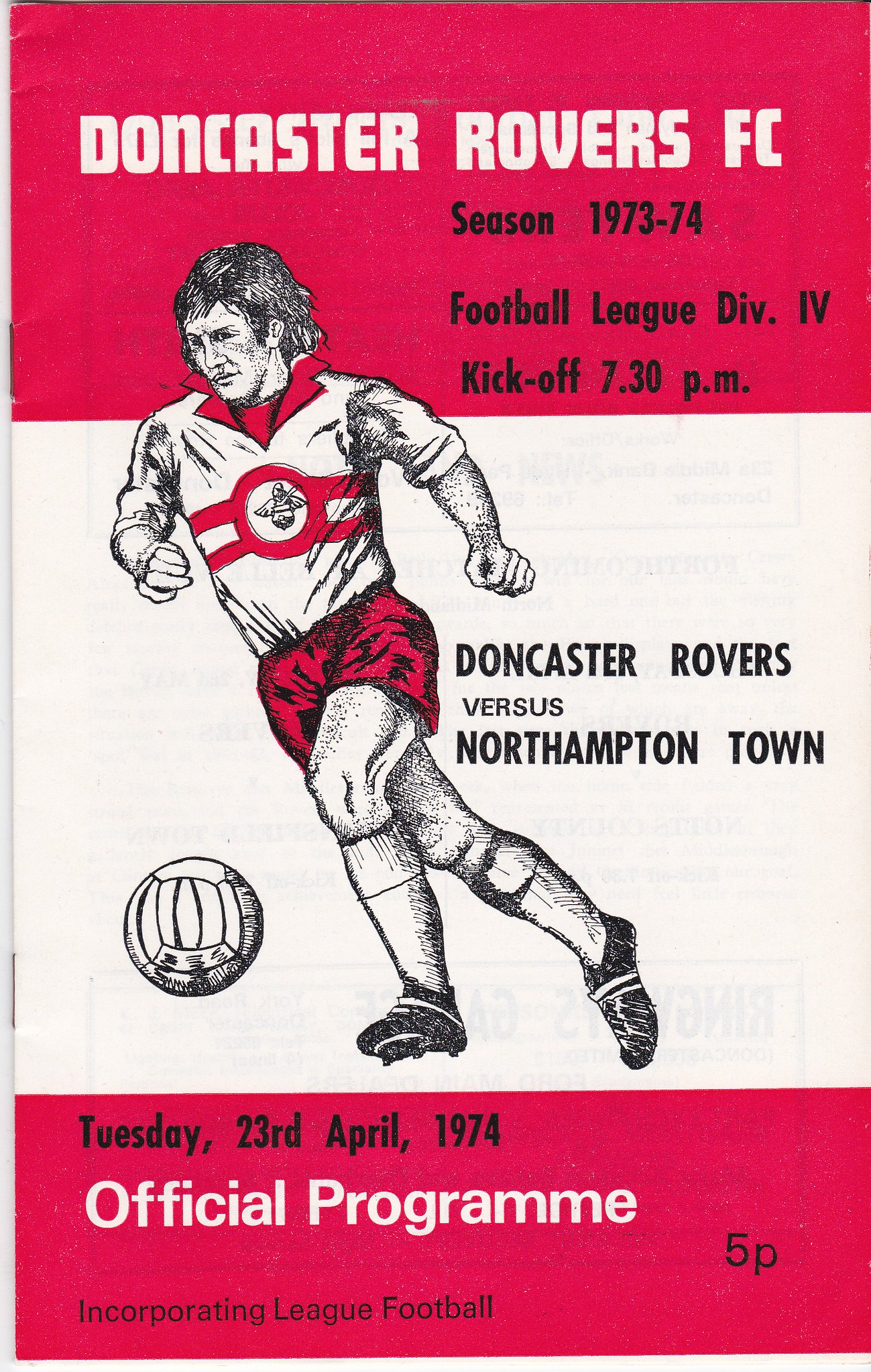The image displays a vintage football program or poster, divided into three color sections: a red rectangle at the top, followed by a white rectangle in the middle, and a red rectangle at the bottom. At the top, a red banner in white capital letters reads "Doncaster Rovers FC." Directly below in black text, it states "Season 1973-1974, Football League Division IV." Further down, it specifies the kickoff time as "7.30 p.m." and then "Doncaster Rovers versus Northampton Town." The central white section features a black-and-white sketch of a male footballer with short dark hair, dressed in red shorts and a red and white jersey, actively chasing a soccer ball. Towards the bottom, in a pinkish banner, the date "Tuesday, 23rd April, 1974" is printed in black. Below that, it reads "Official Program" in large white text, with "5P" to the right. At the very bottom, it mentions "Incorporating League Football" in small black text. The overall color scheme is red and white, consistent both in the background and the footballer's attire.